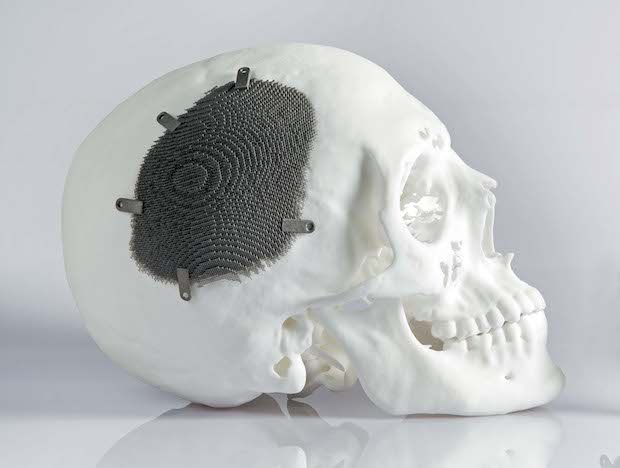The image depicts a white human skull resting on a slightly reflective white surface, set against a neutral white and light grey background. The skull, appearing almost as though it has been bleached, is shown in profile with the face pointing to the right and the back of the skull to the left. The skull features detailed anatomical structures, including visible teeth, jawline, eye sockets, and nasal cavity. The composition is carefully lit, creating light reflections and subtle shadows behind the skull.

Noteworthy is a grey, mesh-like patch on the side of the skull, potentially indicative of a medical application, such as a post-operative or trauma-related repair. This patch, which resembles a 3D-printed structure, is attached to the skull using five small metal clips distributed unevenly around its circumference. The clips, which appear as darker, tab-like elements, securely fasten the mesh to the skull, contouring to its surface. The mesh itself has a textured, grid-like pattern and slightly irregular edges, adding a sense of roughness and intricate detail to the overall sleek and clinical appearance of the image.